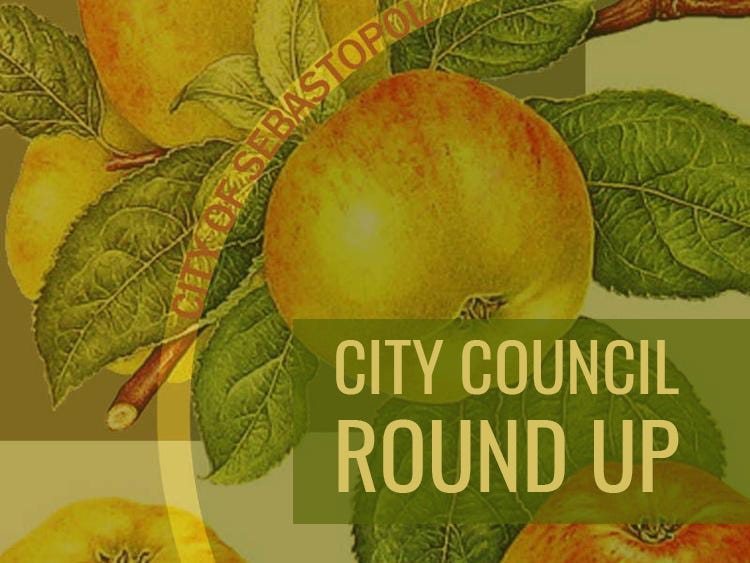This computer-generated image, likely intended for a website or blog, serves as an advertisement for the Sebastopol City Council Roundup. The central focus is a prominently placed apple with green and red streaks, surrounded by leaves, indicating that it's still on the tree. Additional apples are strategically positioned: one in the upper right corner, another just beneath it, one partially visible in the lower right corner, and yet another in the bottom left corner.

The background of the image is mainly green with various shades of brown, highlighting the natural, earthy theme. At the bottom right, a green translucent banner displays the title "City Council Roundup" in bold white letters, drawing immediate attention. To the left of this, another banner in yellow with red text reads "City of Sebastopol," ensuring the viewer knows the originating city. This detailed and vibrant backdrop emphasizes the community-focused event with a visually appealing blend of fruit, foliage, and clear, inviting text.